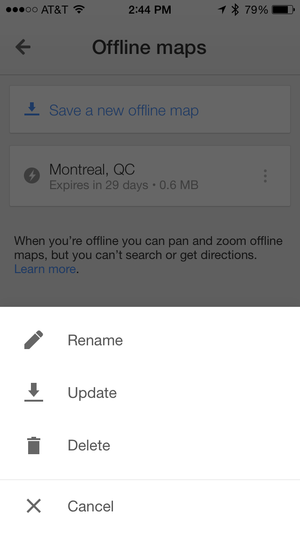The image appears to be a screenshot from a smartphone, displaying a screen from an offline maps application. 

In the top-left corner, the status bar shows three out of five dots filled, indicating signal strength, with 'AT&T' next to it. A Wi-Fi signal icon is present, followed by the time '2:44 PM'. Bluetooth is enabled, as shown by the icon, and the battery percentage is 79% with a corresponding battery icon. 

Below the status bar, the main interface of the offline maps app is visible:
- At the top, the title 'Offline maps' is displayed with a left-facing arrow next to it.
- Below the title, there's an actionable text 'Save new offline map' in blue, accompanied by a clickable button.
- Listed next is an offline map titled 'Montreal QC,' which expires in 29 days and is 0.6 megabytes in size. To the right of this rectangle, three vertically aligned dots suggest more options.
- The screen explains that when you're offline, you can pan and zoom the offline maps, but searching or getting directions is not possible. This is followed by a blue hyperlink 'Learn more'.
  
Further down, there are several options represented by icons and text:
- A pencil icon labeled 'Rename'
- A down-facing arrow with a line (usually indicating download) labeled 'Update'
- A trash can icon labeled 'Delete'
- An 'X' icon labeled 'Cancel'

All text is in gray, except for hyperlinks which are highlighted in blue. The layout is clean and provides functional options for managing offline maps effectively.